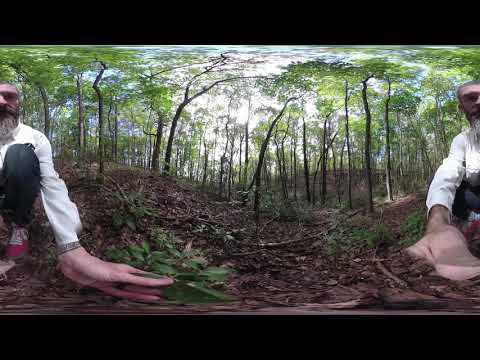The image appears to be a mirrored, slightly distorted photograph taken outdoors in a wooded area, possibly in a forest or rainforest setting. The ground is covered with brown leaves, sticks, and brush, creating a rich, textured layer of forest debris. The scene is set on what seems to be a cliff bank or elevated area with dense, native vegetation. The photo captures a man with a gray beard and mustache, wearing a white and navy blue long-sleeve shirt. He is crouched down and holding a leaf in his hand, presenting it to the camera. Due to the mirrored effect, his image appears on both the left and right sides of the photo, with only half of his body visible on each side. The background features trees and a partly cloudy sky. The overall image has a blurry, watercolor-like effect with colors including black, white, gray, green, brown, and hints of red and pink. There is no text, but black banners are present at the top and bottom of the photo. The dimensions of the image are approximately five inches by four inches tall.